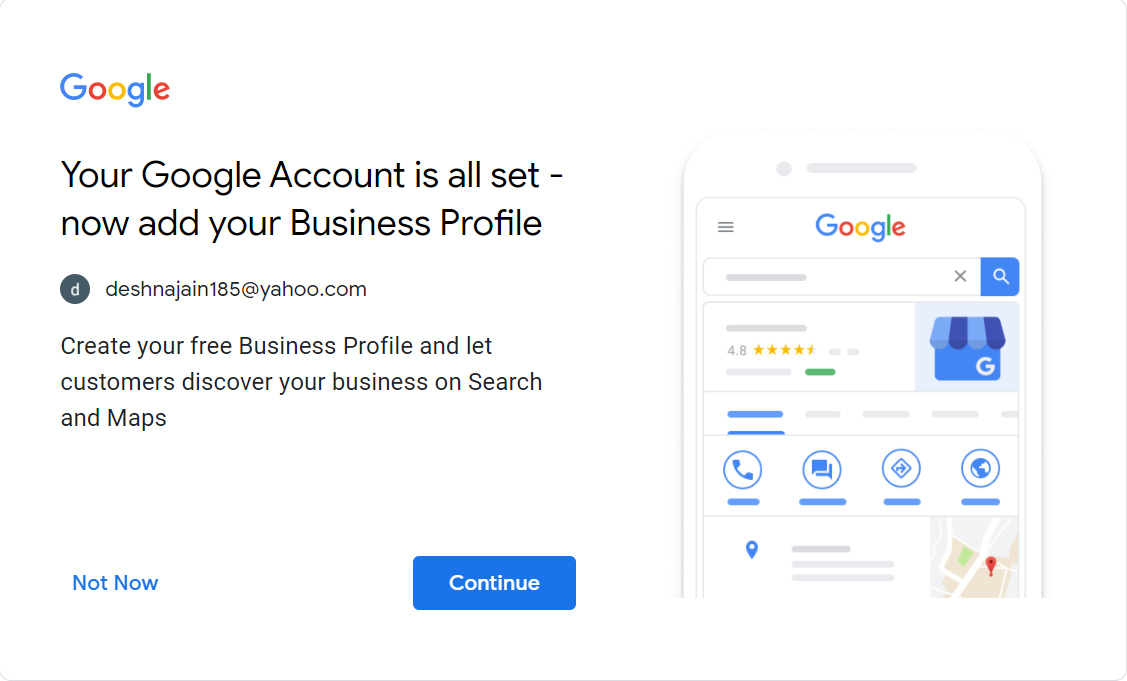Displayed on the screen is an open page from Google. In the upper left corner, the colorful Google logo stands out prominently, while below it, a message in bold black text reads, "Your Google account is all set. Now add your business profile." Directly underneath this message, in smaller gray letters, is the initial "D" encased in a small gray circle, accompanied by the email address "SeanJane185@yahoo.com."

Further down, a larger prompt encourages users to "Create your free Business Profile and let customers discover your business on Search and Maps." At the bottom left corner of the screen, there's a blue button labeled "Not now," and on the opposite side, another blue button reads "Continue."

On the right side of the screen, there is a simplistic outline of a smartphone. Centered at the top of this smartphone illustration, Google is displayed again, followed by a search bar beneath it. Below the search bar, there's a small blue icon resembling a market or house with a "G" inside. Further down, there is a rating of "4.8" accompanied by yellow stars.

Aligned from left to right under the rating are four icons: a phone, a conversation bubble, a share arrow, and an Earth symbol. Below these, a blue location pin icon appears, and across from it, in the lower right corner, there's a red location pin on a small grayed-out square map.